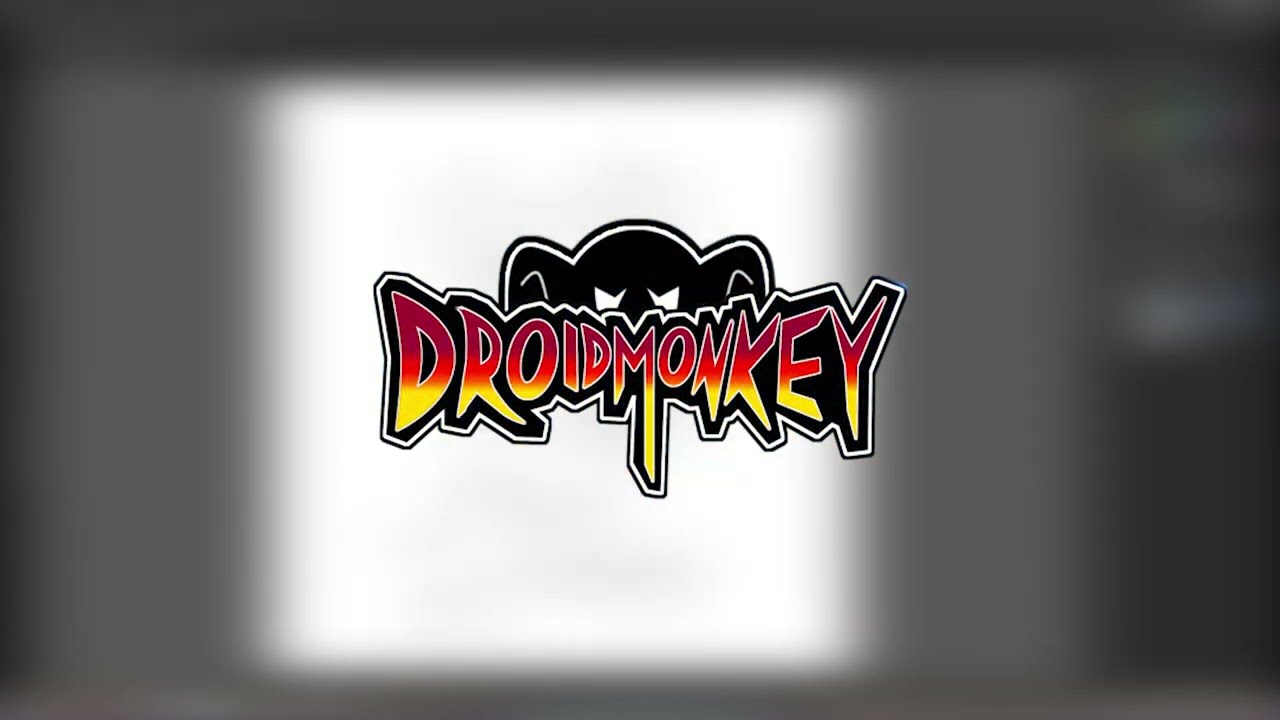The image is designed in a landscape orientation, featuring a centered logo for "Droid Monkey." The logo's text "Droid Monkey" is prominently displayed with a gradient fill transitioning from deep red at the tops of the letters, to orange in the middle, and finally yellow at the bottoms. The letters are intricately outlined: first with a very thin white stripe, then a slightly wider black outline, followed by another thin white stripe, and finished with a very thin black outline, adding dimension to the text.

Above the center of the text is the upper head of a monkey, rendered in solid black with striking white eyes that give it an angry appearance. The monkey head also features an outline sequence similar to the text: thin white, followed by black, echoing the layered outlining effect. 

The background is a blurred, possibly digital workspace environment, heavily unfocused and mostly indistinguishable. It consists of several rectangular shapes in varying shades of gray, with a glowing white square block immediately behind the main logo, further framed by lighter and darker gray rectangles. On the far right side of the background, there are blurry hints of green, yellow, and blue lights, likely part of the digital workspace interface. The overall logo embodies a bold and edgy aesthetic, with the words "Droid" and "Monkey" closely positioned and styled with jagged, chaotic letterforms.